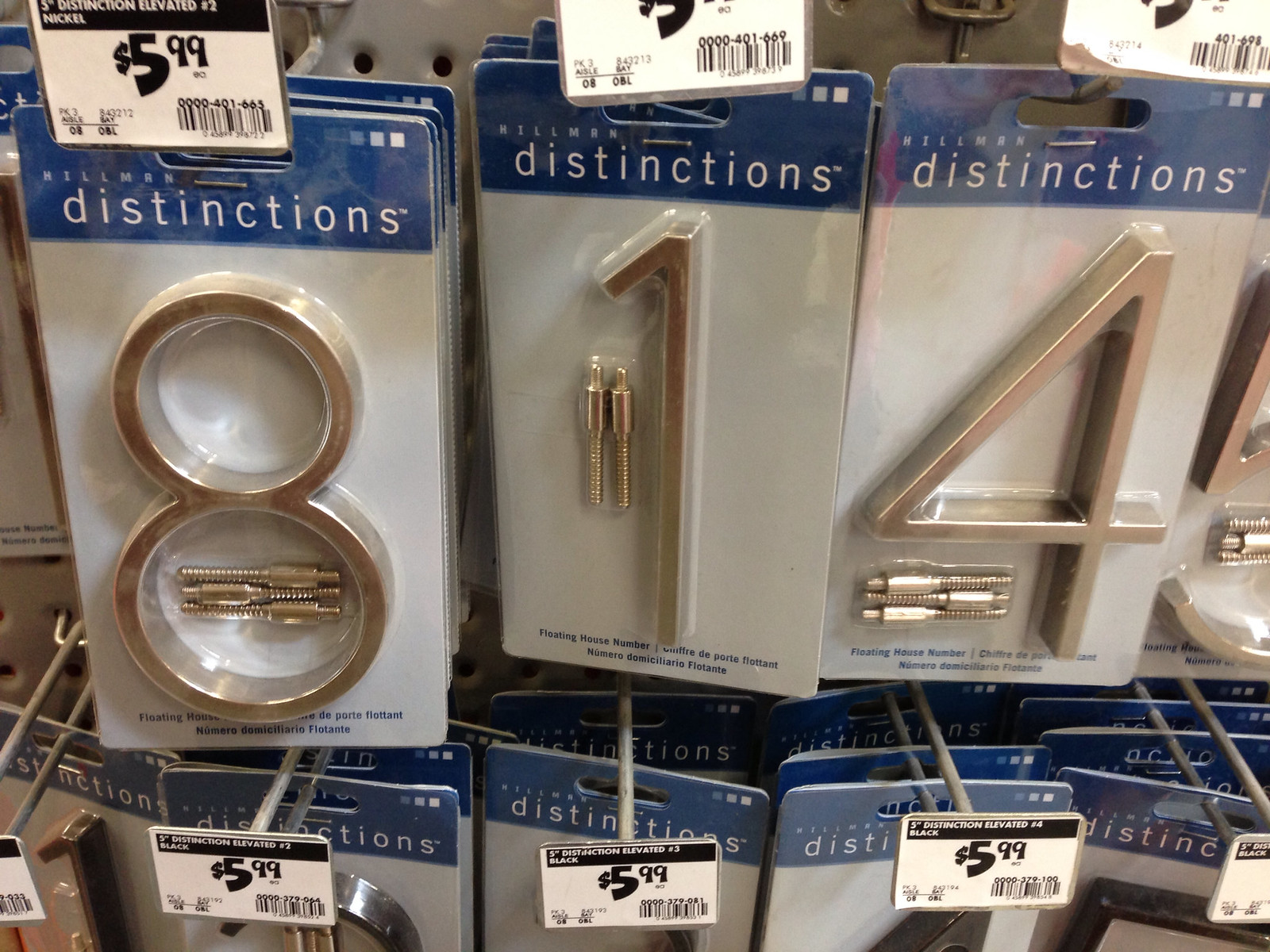This photograph, likely taken in a Lowe's or Home Depot, captures a well-organized aisle dedicated to house letters and mailbox numbers. Prominently displayed are large brass-colored house numbers, each approximately 8 inches in height. Visible numbers include 8, 1, 4, and 5, while lower shelves feature black and silver-colored numbers such as 2 and another 4. Each number is priced at $5.99 and comes with the necessary mounting hardware. The assortment suggests the availability of various sizes, colors, and possibly different styles within the aisle. The presentation reflects a good value for high-quality, durable house numbers.